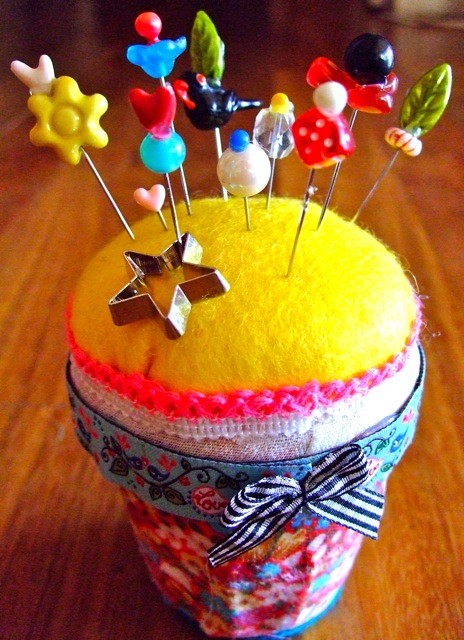This image depicts a vibrant and intricately designed pincushion that resembles a small flower pot. The pincushion is covered with layers of colorful fabric: at the top, a bright yellow felt material, followed by layers of pink, white, and a flowery red, blue, and orange pattern at the bottom. Encircling the pincushion is a decorative blue and white striped bow.

The top yellow portion of the pincushion is adorned with a variety of unique and interesting pins, at least ten in number. Each pin features a distinct and collectible design: a red dice, two green leaves, a white circle, a blue circle with a red heart, a pink heart, a yellow flower, and a metal star, among other shapes like birds.

The pincushion itself is highly decorative, with an additional row of lace and rickrack accents—pink at the very top and white below it—adding to its charm. The fabric surrounding the pot includes bright colors like blues, pinks, whites, and a bit of lavender, complemented by ivy leaves and swirling red floral patterns on the ribbon. Overall, this pincushion is not only a practical tool for knitters and sewers but also a beautiful and collectible piece of craftsmanship.